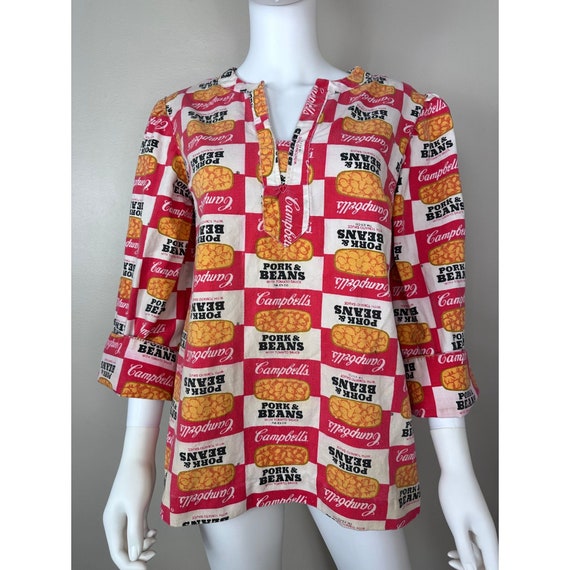This color photograph features a white headless mannequin standing in front of a gray wall, modeling a mini dress that reaches mid-thigh. The mannequin's legs are visible below the dress, and its hands are positioned by its sides. The dress has long sleeves that extend halfway down the forearms, an open collar, and a V-line zipper that runs partway down the front. The fabric of the dress is adorned with a repeating pattern of Campbell's Pork and Beans labels. Each label consists of a red top section with "Campbell's" written in white text, an image of pork and beans in the middle, and a white bottom section with the words "Pork and Beans" in black text. The detailed design gives the dress a unique and visually engaging appearance reminiscent of the iconic Campbell's soup cans.